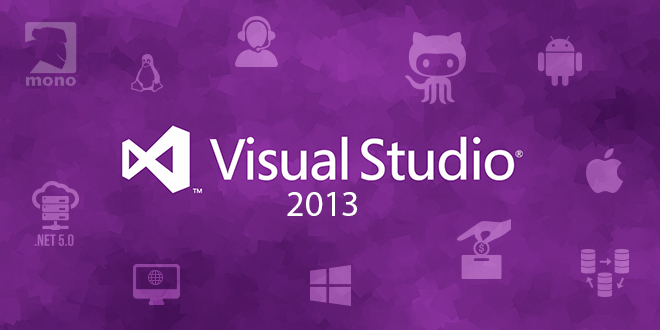The image features a rectangular screen with a dynamic, faux finish in various shades of purple and lavender. Deep purples merge seamlessly with lighter and medium tones, creating a rich, textured backdrop. Centrally placed in bold, white block text are the words "Visual Studio," with "2013" positioned directly beneath. To the left of the text, a white bow-like logo represents the Visual Studio brand. The screen is further adorned with faint icons in a pale lavender shade, subtly enhancing the background. On the lower left, a computer monitor icon is visible, followed by the Windows logo to its right, and a hand inserting a coin into a box further along. On the center-right, an apple icon stands out, while the upper-right area features the familiar Reddit character, resembling a small robot.